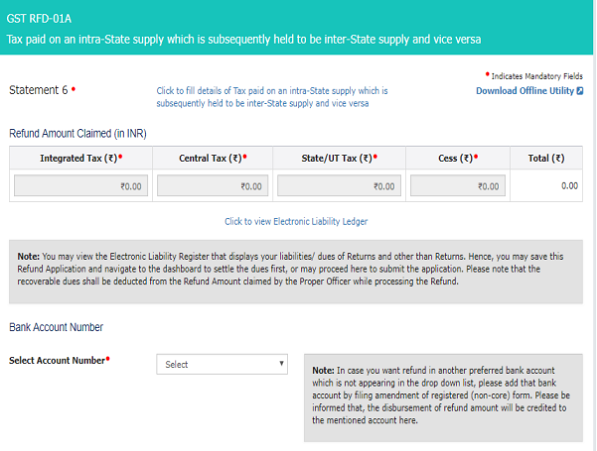The image depicts a section of a billing statement interface for tax services. At the top, there's a teal green colored bar with white text that reads "GST-RFD-01A." Below this, the text explains that the form is for "tax paid on an intrastate supply which is subsequently held to be interstate supply and vice versa." Beneath this bar, a white background section contains the heading "Statement 6."

Further down, there's blue text prompting the user to "click to fill details of a tax paid on interstate supply which is subsequently held to be interstate supply and vice versa." To the right of this prompt, an option to "download offline utility" is visible. The section also includes fields to claim a refund amount in Indian Rupees (INR) for different tax categories: Integrated Tax, Central Tax, State/UT Tax, Cess, and the Total. Each of these fields has a rupee symbol next to its title and currently displays a value of zero.